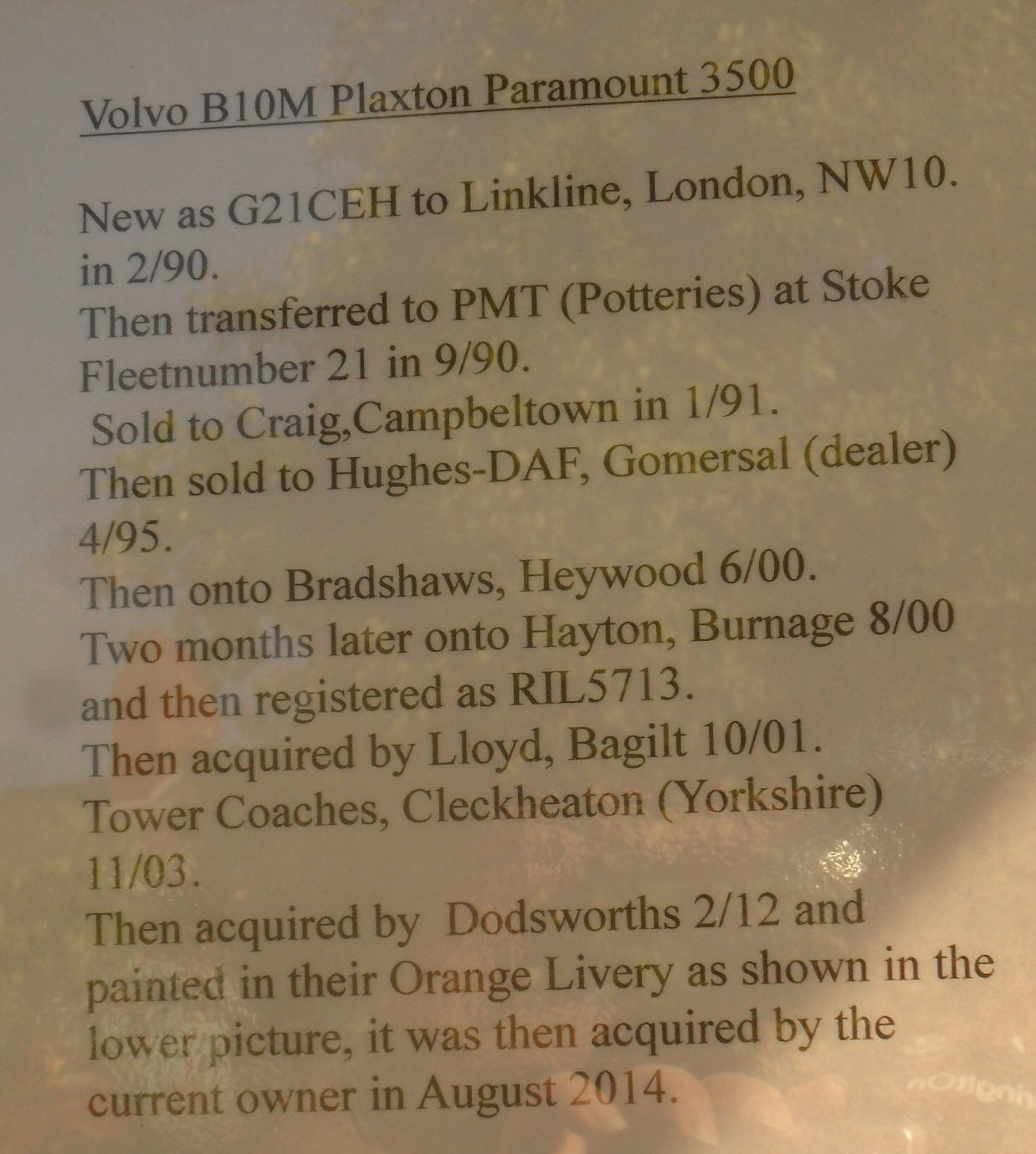The image shows a typed document on a white piece of paper detailing the history of a vehicle, Volvo B10M Plaxton Paramount 3500, with the title underlined at the top. The text provides a chronological account of the vehicle's ownership and registration: initially new as G21CEH to Linkline London NW10 in February 1990, then transferred to PMT Potteries at Stoke, Fleet Number 21, in September 1990. It was sold to Craig in Campbeltown in January 1991, then to Hughes DAF Gomersall Dealer in April 1995, followed by Bradshaw’s Haywood in June 2000. Two months later, it went to Hayton Burnidge in August 2000 and was registered as RIL5713. It was acquired by Lloyd Bagulett in October 2001, transferred to Tower Coaches in Cleckheaton, Yorkshire in November 2003, and later acquired by Doddsworth in December 2012, where it was painted in their orange livery as the lower picture shows. The current owner acquired it in August 2014. Reflections of a tree, a person's face, and hands are also visible on the page, giving an additional layer of detail to the document.